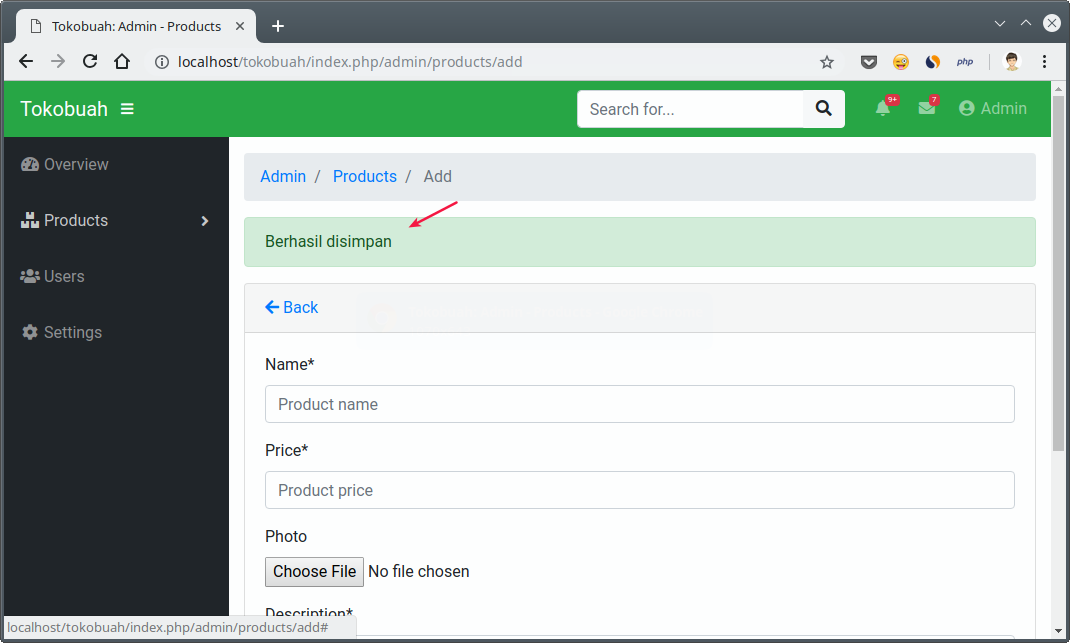In this screenshot, we are viewing the upper left-hand corner of a browser window or tab named "Tokobuwa Admin Products." The URL shown in the address bar reads "localhost//tokobuwa//index.php//admin//products//ad." On the left side of this interface, there is a vertical black navigation bar under the "Tokobuwa" header, featuring the options: Overview, Products, Users, and Settings.

Prominently in the center of the screen, displayed within a large white rectangular section, the top line reads "Admin//Products//Ad." Below this, in a light green box, is the text "Berhazel Disenpan," followed by a blue hyperlink labeled "back."

Within the main white content area, there are two text input boxes. The first is labeled "Name," and contains the placeholder text "Product Name." The second box is labeled "Price," with the placeholder "Product Price." Additionally, there is an option for "Photo" followed by a button labeled "Choose Photo."